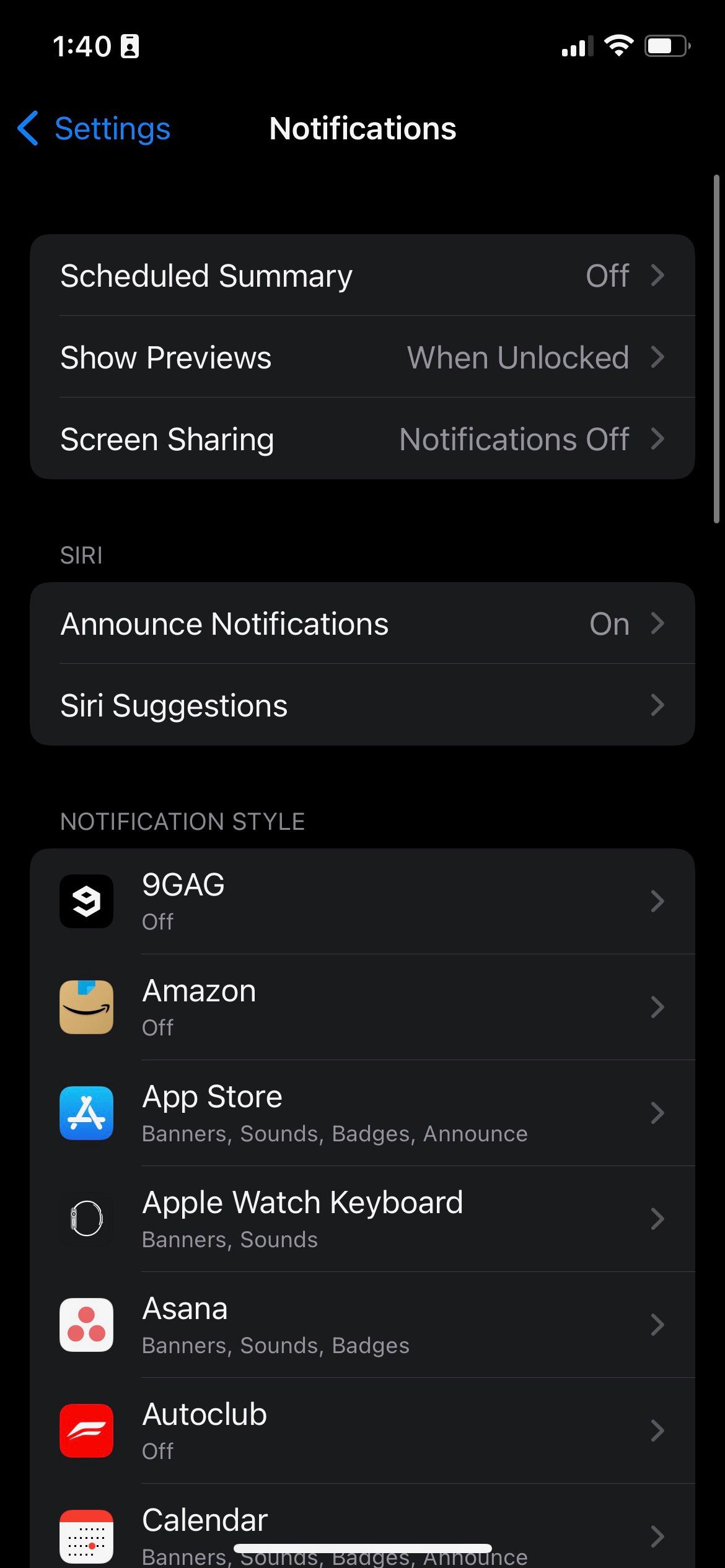This screenshot captures the notification settings screen of a smartphone. The interface features a black background with three sections displayed on dark gray panels.

At the top of the screen, the title "Notifications" is prominently displayed. To its left, a blue back arrow appears, indicating a way to return to the previous screen.

The first section lists three options with a gray background and white text: "Scheduled Summary," "Show Previews," and "Screen Sharing."

The second section is labeled "Siri." Within this section, there are options for "Announce Notifications" and "Siri Suggestions."

Following the Siri section, there is a "Notification Style" category showcasing how various apps manage notifications. This list displays several apps along with their notification statuses:
- 9GAG: Off
- Amazon: Off
- App Store: Banner, Sounds, Badges, Announce
- Apple Watch: Notifications
- Keyboard: Notifications
- Asana: Notifications
- Auto Club: Notifications
- Calendar: Notifications